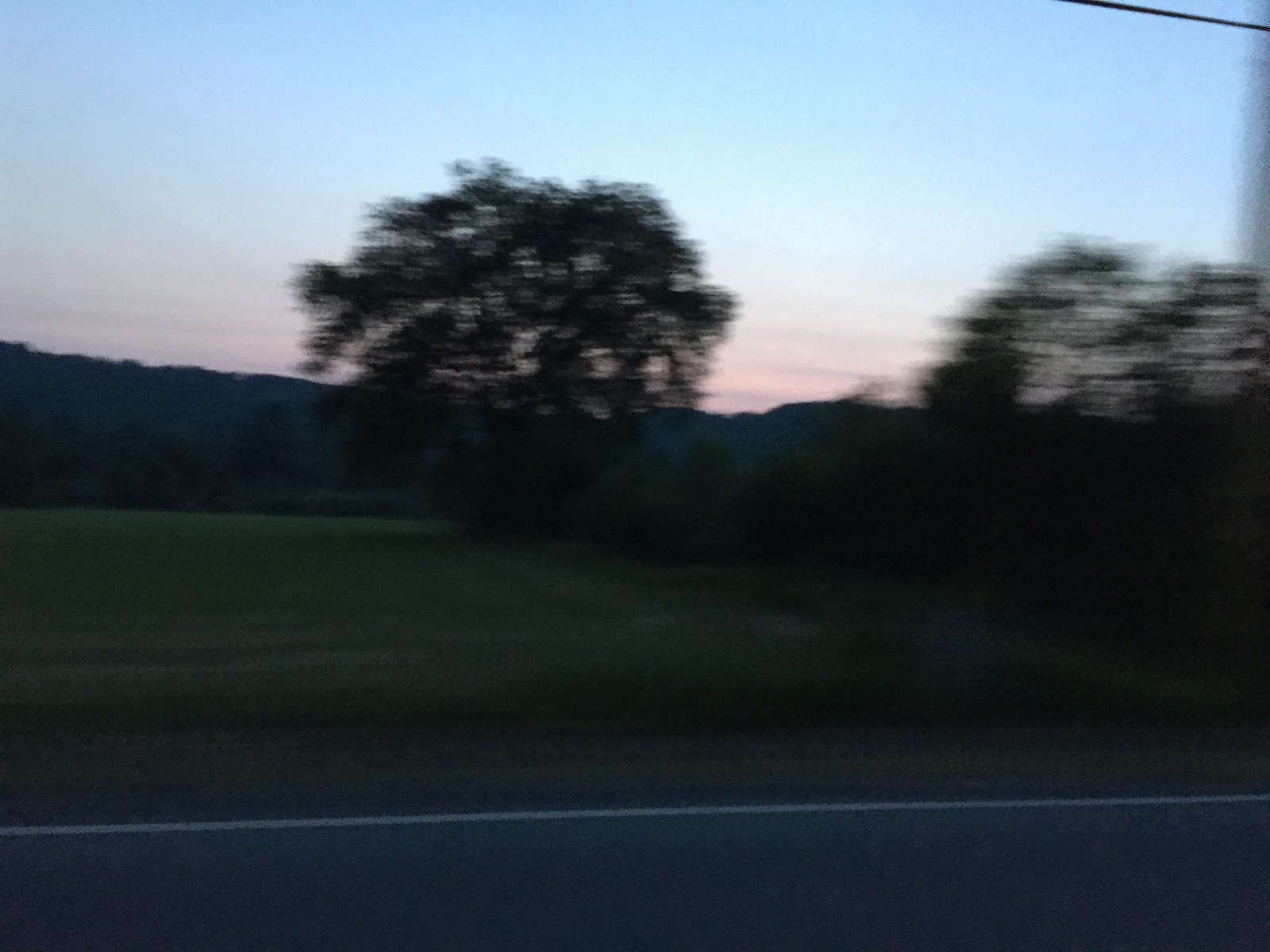The photograph, taken from inside a moving car at dusk or just after sunset, captures a rural scene with a horizontal road at the bottom, marked by a white line along its edge and a dirt shoulder. A green meadow stretches out beyond the road, featuring a large tree and partially silhouetted by the fading light. In the distance, dark, wooded hills create a soft horizon under a sky transitioning from reddish-pink near the horizon to a deeper blue higher up, accentuated by scattered clouds. The foreground includes what appear to be oak trees, their green canopies blurry due to the motion of the car, making them challenging to detail. A single power line is faintly visible in the upper right corner of the image, adding to the sense of motion and the twilight atmosphere.